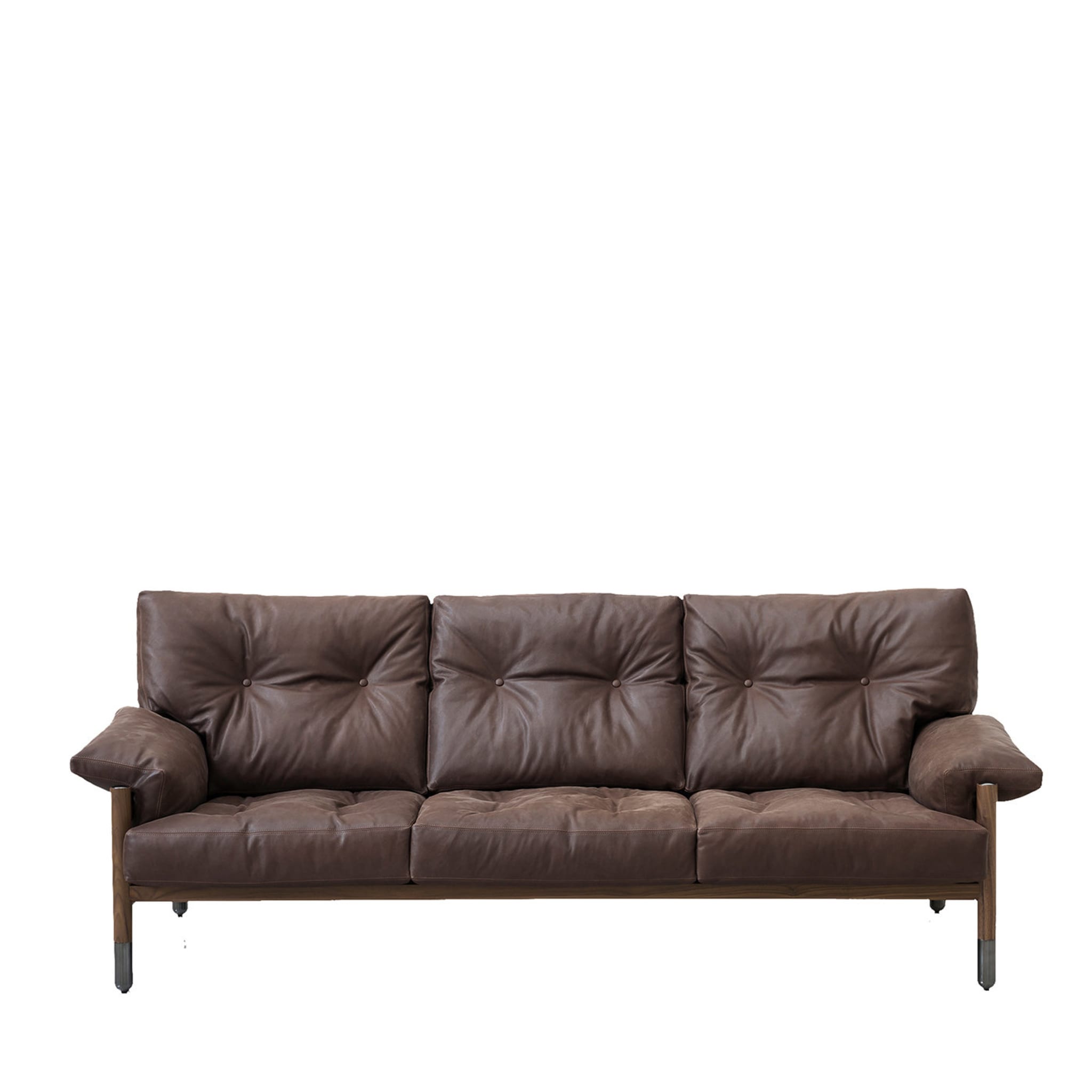This image presents a detailed view of a three-seater brown leather couch, set against a white background. The couch rests on slender wooden legs, reminiscent of pencil legs, creating an elegant but simple design. The seat and backrest cushions are well-worn, featuring visible ridges that mark familiar use. Each seat cushion is approximately three inches thick and tufted with brown buttons, lending a classic dimpled appearance to the furniture. The wrapped cushions that form the armrests add to the overall comfort and aesthetic. The piece appears to be constructed with a wooden frame supporting both the structure and the cushions. Its dimensions and layout suggest it comfortably seats three people and spans about seven feet in length. The setting is minimalist, with no floor visible, highlighting the couch against the white background as if for a catalog or online furniture preview. The detailed photograph captures the inviting softness and practical design of the couch, making it seem like a cozy yet stylish addition to any living space.